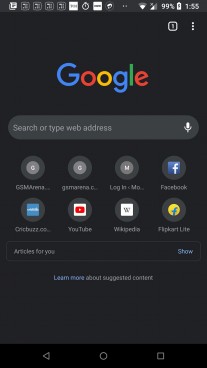The image showcases the Google home page on a mobile phone. The top section features a gray border containing various app icons, predominantly square-shaped, with one circular icon resembling a clock. In the upper-right corner, the Wi-Fi and data icons are both shown as half filled. Adjacent to these icons, the battery icon indicates a 99% charge, accompanied by a charging symbol, and the time is displayed as 1:55. Just below this section, a white three-vertical-dots icon for more options appears against a black background.

Center stage, the Google logo is prominently displayed with its signature colors—both Gs in blue, the first O and the E in red, the second O in yellow, and the L in green. Directly beneath, there's a search bar with the placeholder text "Search or type web address," accompanied by a microphone icon for voice search.

Further down, the screen presents eight panels of frequently viewed pages, which include GSM Arena, a Facebook login page, Chick Buzz, YouTube, Wikipedia, and Flipkart Lite. There are also sections labeled "Articles for you," "Show," and "Learn more about suggested content."